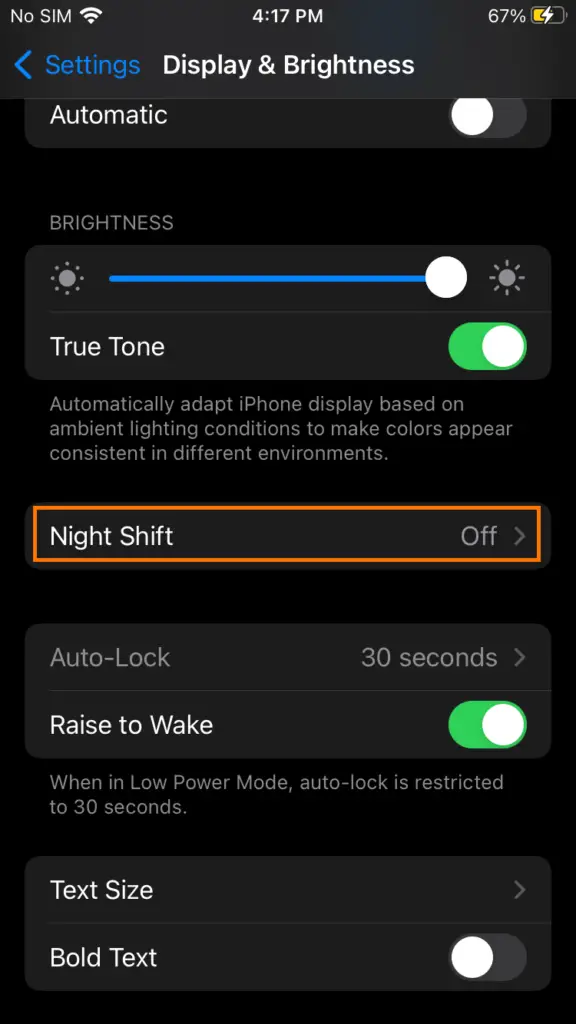The image depicts a screenshot of an iPhone's "Display & Brightness" settings, with the background set to black. At the top of the screenshot, the status bar shows "No SIM card," the time as 4:17 PM, and the battery level at 46%, currently charging. Directly beneath the status bar is the "Settings" title, alongside the "Display & Brightness" sub-menu title.

Within the "Display & Brightness" settings, several toggles and options are visible:

1. **Appearance:** 
   - **Automatic:** The option is set to off, meaning the iPhone does not automatically switch between light and dark mode.

2. **Brightness:**
   - The brightness slider is set to maximum.
   
3. **True Tone:**
   - This feature is toggled on, allowing the display to automatically adapt based on ambient lighting conditions to maintain color consistency in different environments. A short paragraph explains this feature: "Automatically adapt iPhone display based on ambient lighting conditions to make colors appear consistent in different environments."

4. **Night Shift:**
   - This feature is currently turned off, and an orange circle highlights it.

5. **Auto-Lock:**
   - Set to 30 seconds, ensuring the screen will lock if inactive for this duration.
   - Below this setting is a note: "When in Low Power Mode, Auto-Lock is restricted to 30 seconds."

6. **Raise to Wake:**
   - This option is toggled on, allowing the screen to turn on when the iPhone is raised.

7. **Text Size:**
   - An arrow indicates more settings are available by tapping this option.

8. **Bold Text:**
   - This feature is turned off.

The toggle switches within this menu are green when on and gray when off, indicating the current status of each setting.